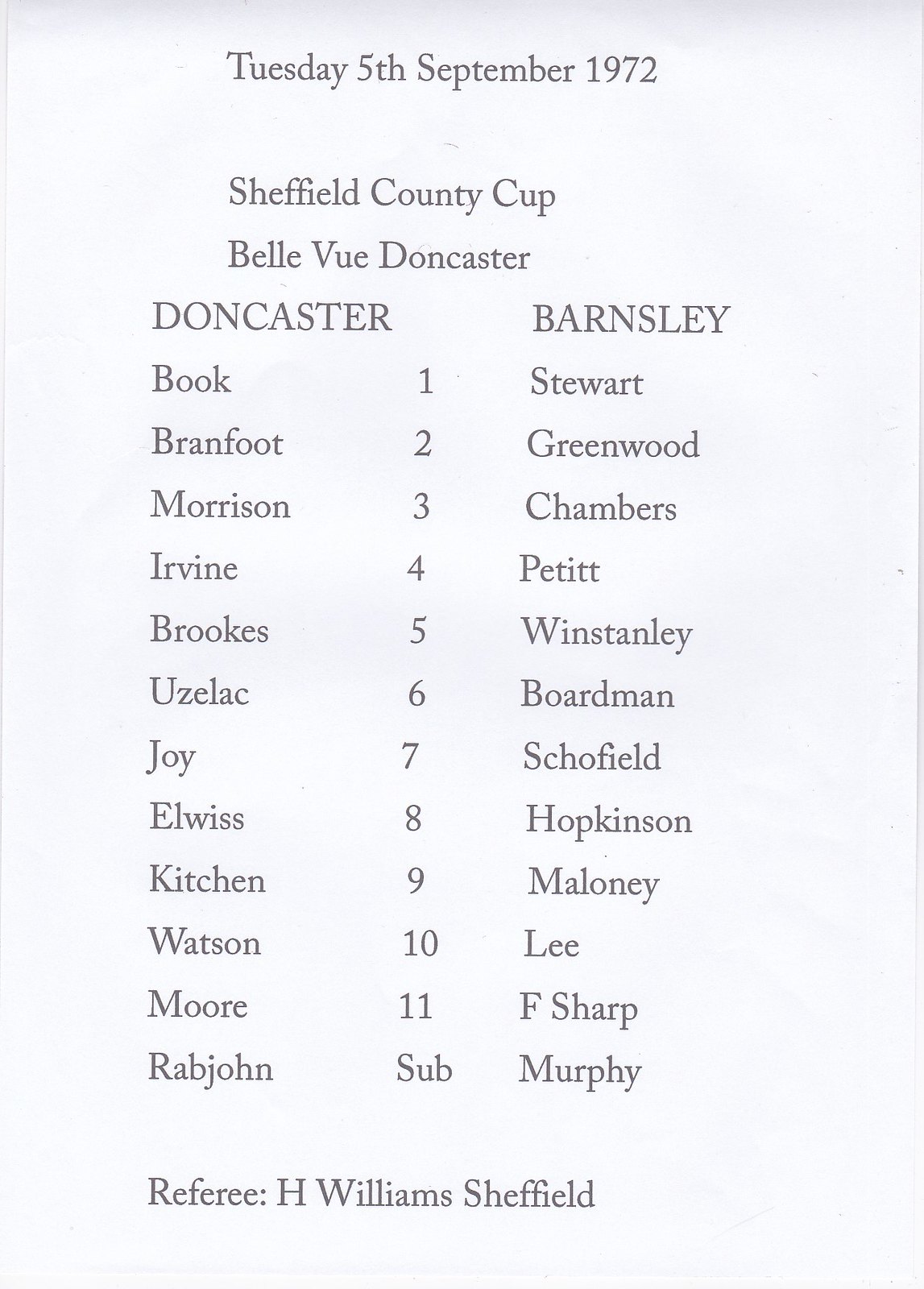The image is a simple, unadorned sports card printed on white paper with black lettering. At the top, it prominently displays "Tuesday, 5th September 1972" and "Sheffield County Cup," followed by "Bellevue Doncaster." The card details a football match between Doncaster and Barnsley, listing the players' names and positions from 1 to 11, with the final entry for each team noted as a substitute. On the left side of the card are the Doncaster players, and on the right are the Barnsley players. Down the middle column, the numbers corresponding to each position are listed. At the bottom of the card, it identifies the referee as H. Williams Sheffield. The design is straightforward, focusing solely on the textual information without any graphics.